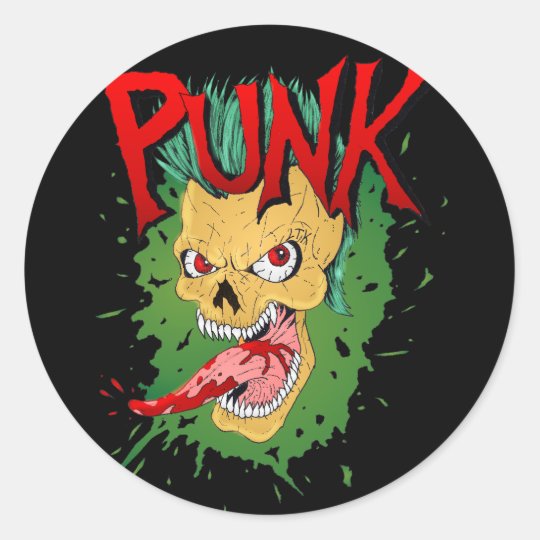The image features a graphic with a white square background and a black circular center. In the middle of the black circle is a striking, yellow skull with a grotesque grin, showcasing many sharp teeth and a long pink tongue covered in blood splats hanging out of the mouth. The skull has vivid, cracked red eyes, and an arch-shaped hole for the nose. It is adorned with a greenish-teal mohawk that extends from the top down the back of the skull. Surrounding the skull is a splash of dark green, resembling paint splatter. At the top of the skull, across the forehead, the word "PUNK" is prominently displayed in big, jagged red letters.